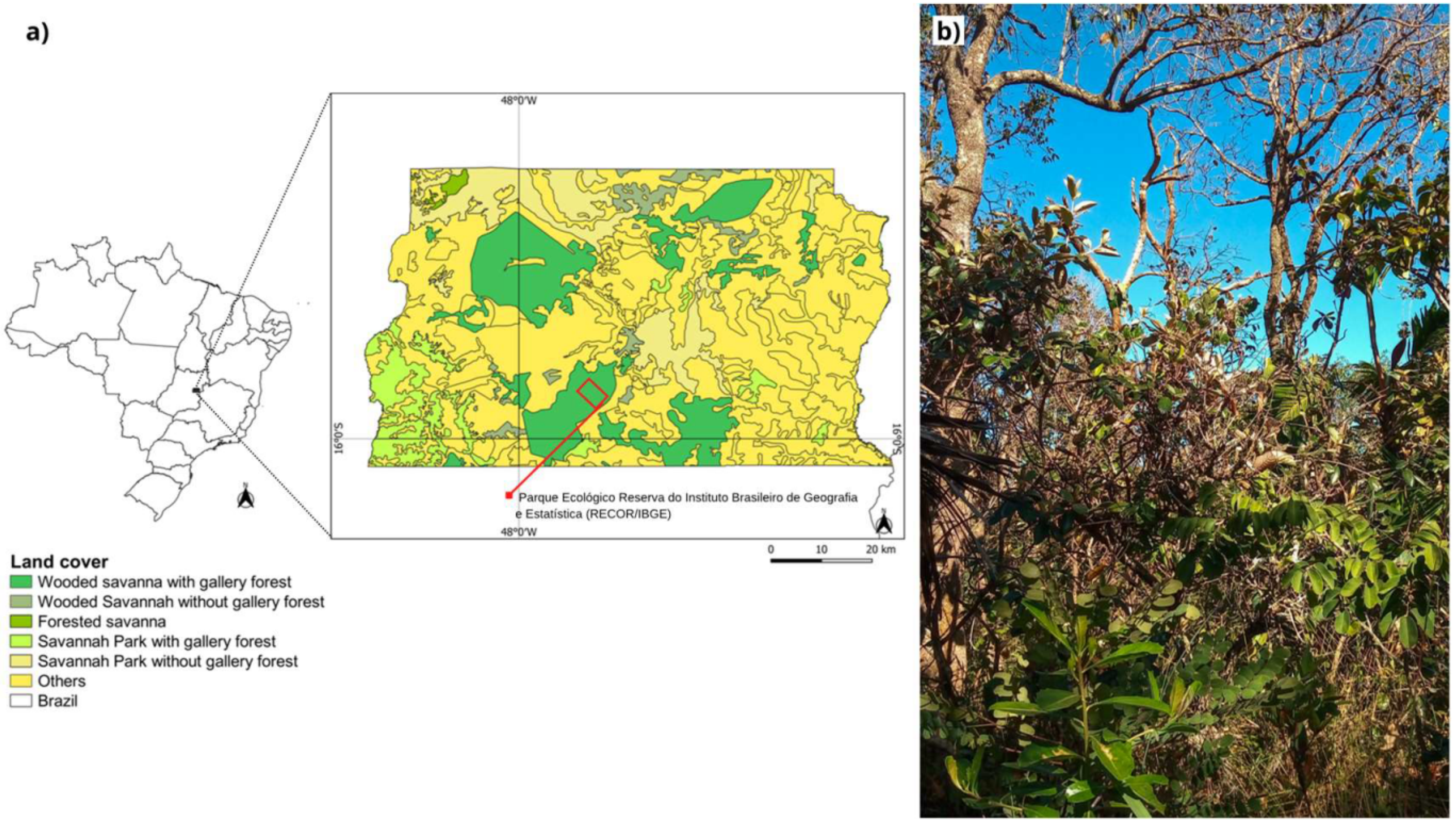This poster illustrates a detailed overview of a forested area within a specific region in Brazil. It is composed of three distinct sections. On the left, there is a simplistic black-and-white lined map of Brazil, alongside a color-coded legend labeled "land cover." This legend explains various forest cover types, progressing from dark green to white: dark green signifies wooded savanna with gallery forest, lighter greens denote different types of savanna, yellow marks savanna park regions, and white represents Brazil. The center of the poster features a zoomed-in, more detailed map of the highlighted region, with green and yellow shades that correspond to the land cover types outlined in the legend. This map includes a scale for distance and a compass for orientation, although the small text below is illegible. The rightmost part of the poster presents an actual photograph of the forested area, showcasing a vivid, crystal-clear blue sky and varying vegetation in shades of brown, gray, and green, with some dead branches reaching skyward. In the top left corner of this photo, there is a small white square marked with the letters 'B' and 'J,' possibly a reference or marker. This comprehensive illustration provides a scientific and geographic portrayal of the land cover in this segment of the Parque Ecológico Reserva in Brazil.